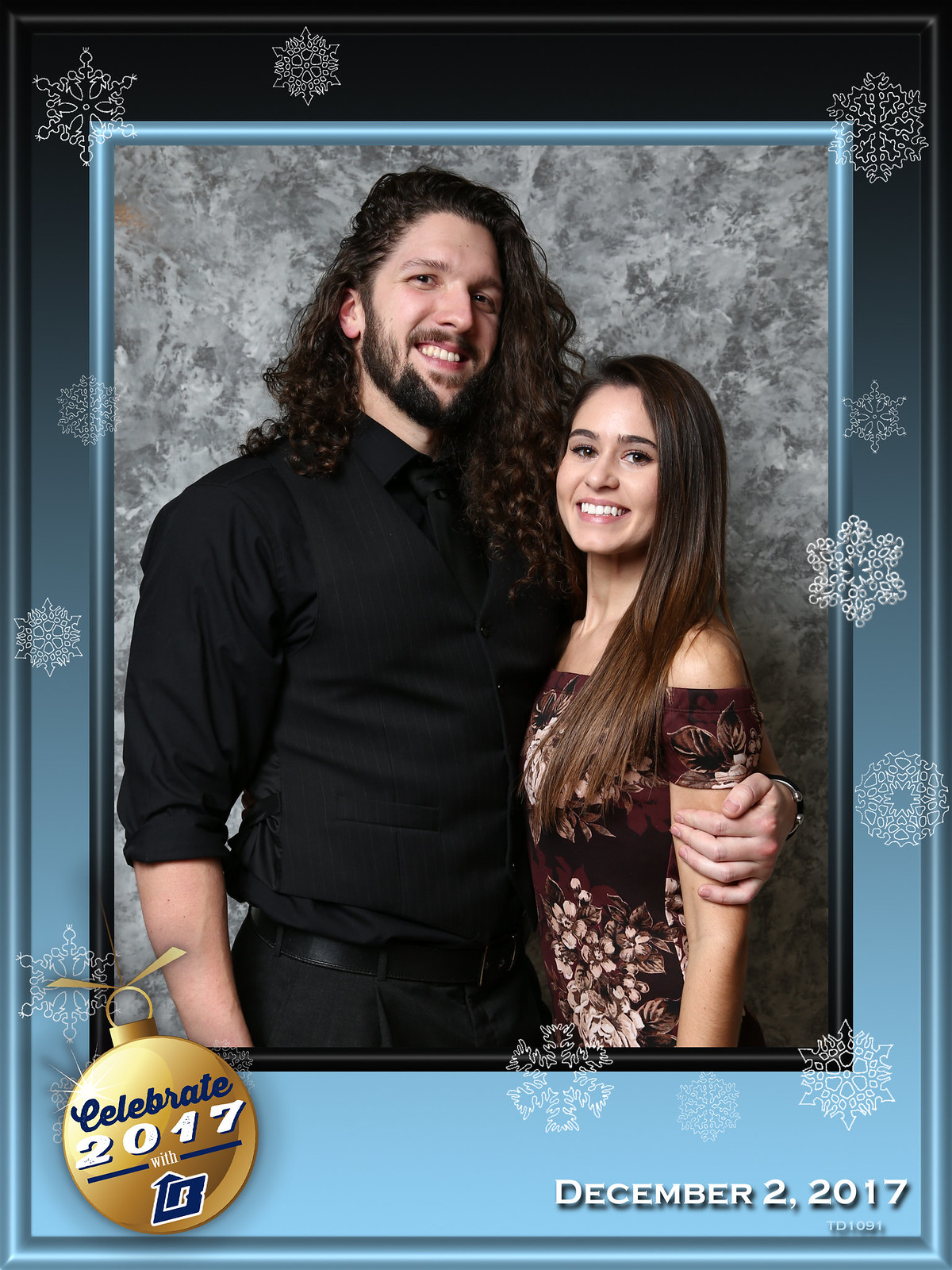The photograph captures a happy couple posing for a holiday card dated December 2, 2017. The tall man on the left has long, curly, black hair cascading past his shoulders, along with a black beard and mustache. He has an olive complexion and is dressed in a black button-down shirt, black pants, and a black belt. His arm is affectionately wrapped around his much shorter partner on the right, who has long, straight brunette hair. She’s wearing a brown floral dress adorned with white flowers. Both are smiling and looking forward. The image is framed with a computer-generated design featuring white snowflakes on the outer edges. In the bottom left corner, a Christmas ornament graphic reads "Celebrate 2017" with a bee logo. The bottom right corner displays the date, December 2, 2017, against a beautifully decorated backdrop meant to evoke a snowy, festive atmosphere.